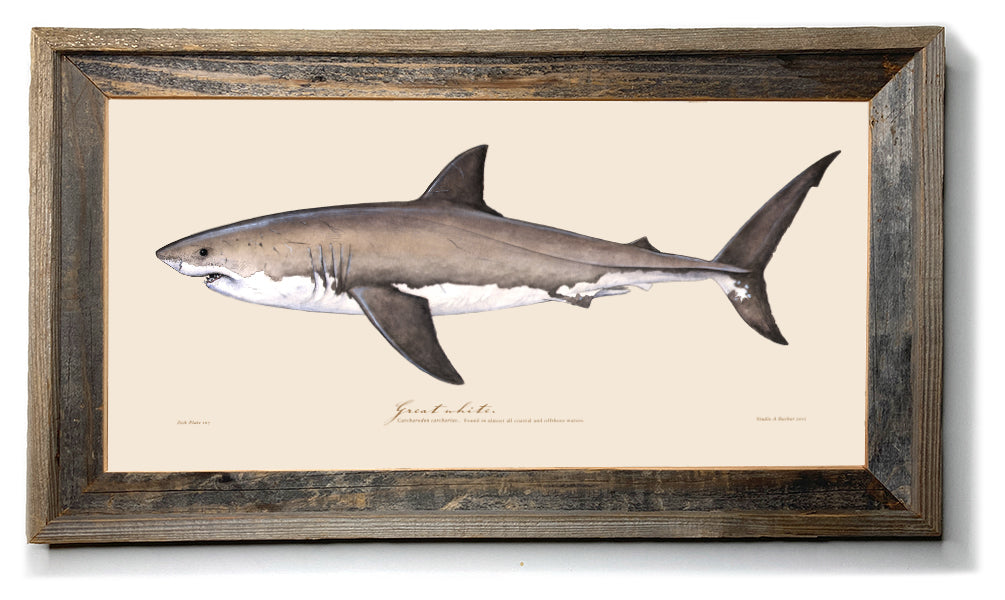This image displays a detailed and realistic drawing or painting of a shark, framed in a rectangular wooden frame with a beveled design. The frame is made of reclaimed wood, featuring a medium brown top level with a sunken area in a grayish-brown hue. The shark, which appears to be swimming towards the left side of the image, is depicted with a white underbelly, a light tan or gray top surface, and dark brown fins and tail. Its open mouth reveals small teeth, and the gills are visible on the side of its body. The background of the artwork is an off-white color. Beneath the shark, there is some text, which includes the words "great white," even though it may not necessarily resemble a great white shark exclusively. The overall dimensions of the framed piece are roughly 18 inches by 24 inches.